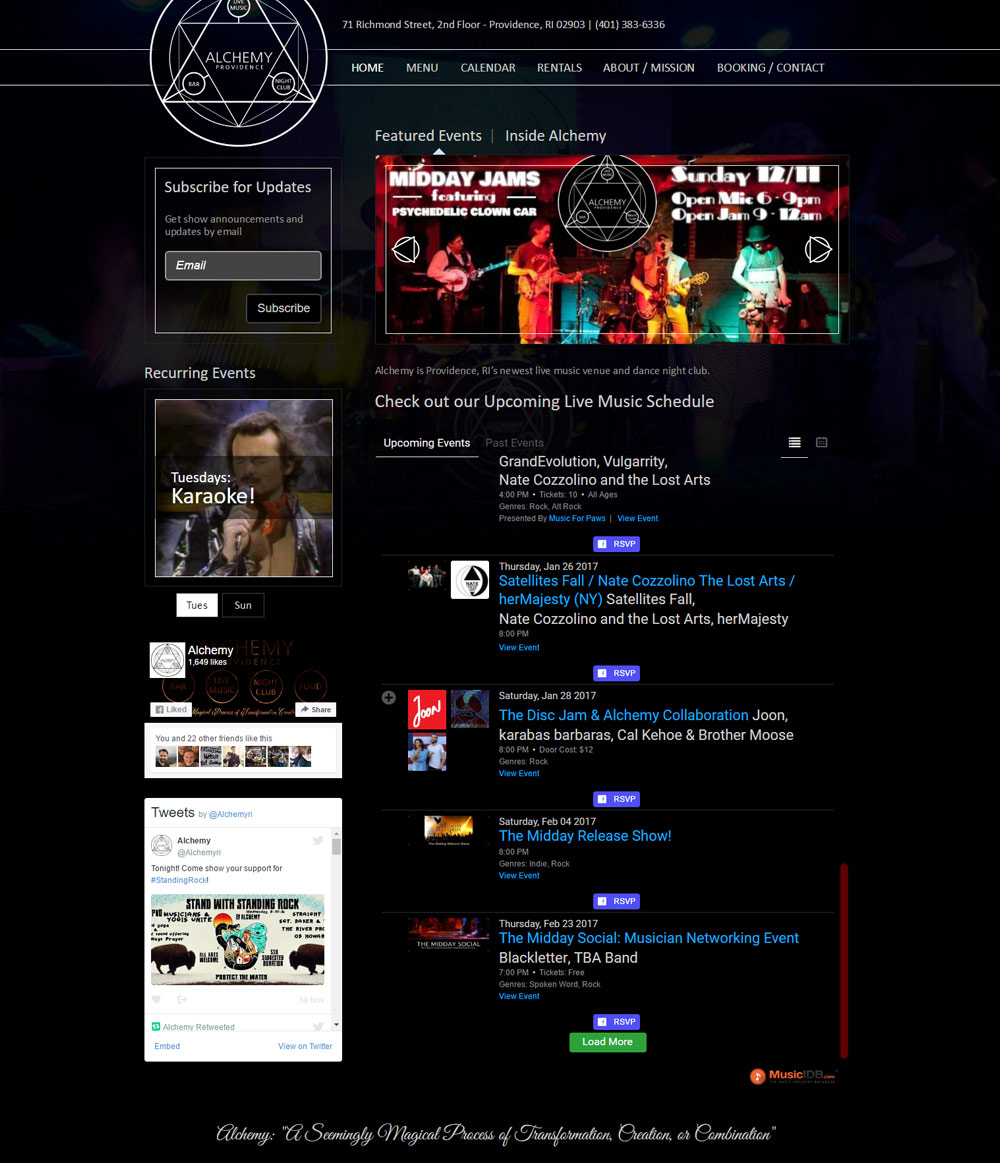The webpage for Alchemy Providence features a sleek, predominantly black design with subtle, muted colors at the top quarter, possibly suggesting a stage backdrop. The rest of the page is entirely black, emphasizing its minimalist aesthetic. In the upper left-hand corner, the logo for Alchemy Providence is prominently displayed. The logo consists of an upright and an inverted triangle intersecting to create a star pattern, encircled by additional decorative elements, all rendered in white font.

The main focus of the webpage is a "Featured Events" section, centered prominently. The events listed include midday performances by Psychedelic Clone Car, as well as other upcoming acts like Satellite, It's Fall, and Nate Cozzolino and The Lost Arts. Each event entry includes specific dates and times, with clickable links for ticket purchases. The website advertises its location as a club situated on the second floor of a building on Richmond Street in Providence, Rhode Island.